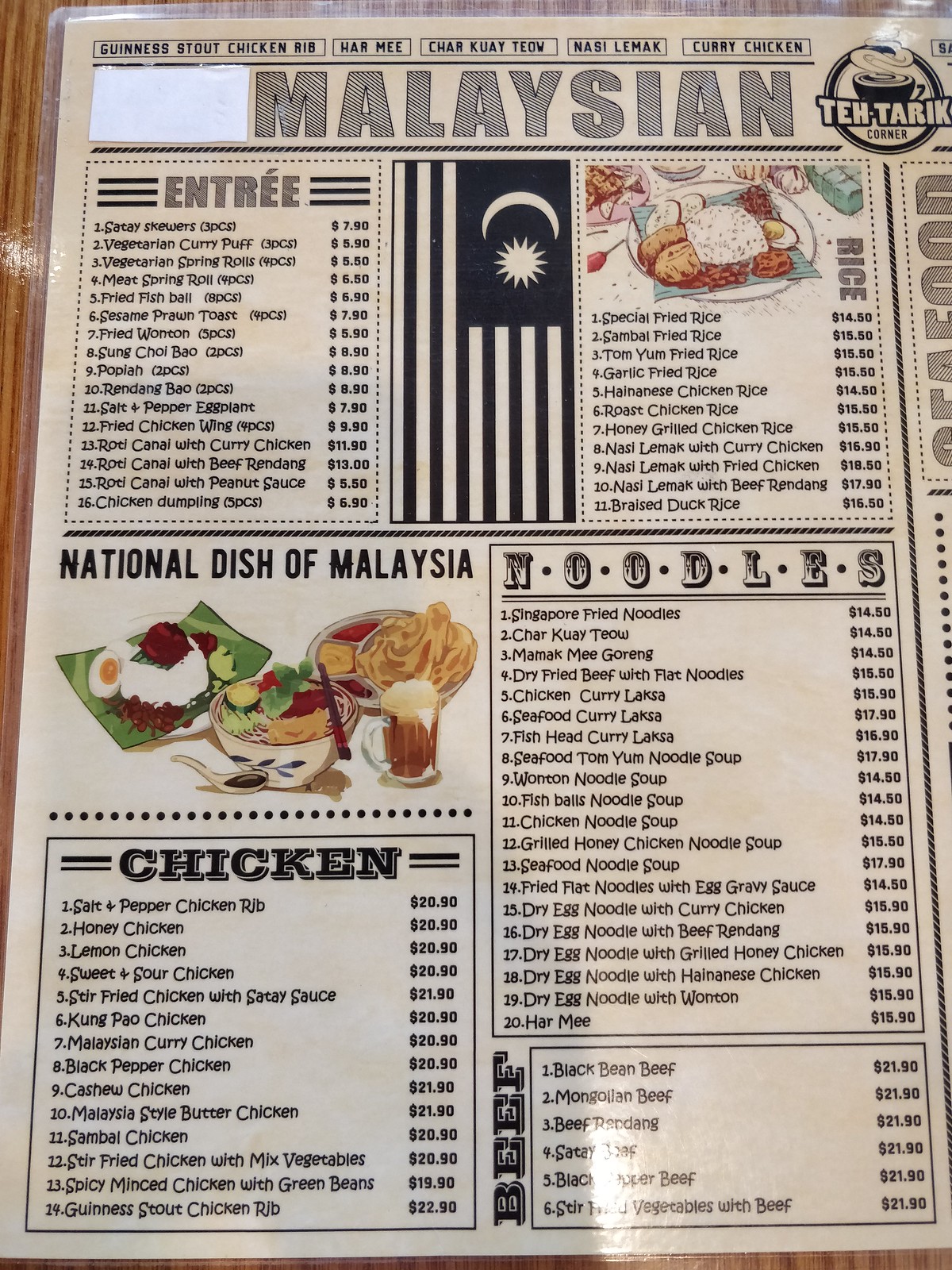The image showcases a detailed menu for Malaysian cuisine from an establishment named Teh Tarik Corner, prominently displayed in the top right-hand corner. The menu is organized into several sections for easy browsing. At the top portion, entrees are listed, providing a variety of options. The middle section highlights Malaysia's National Dish, giving it special emphasis. Below, there's a dedicated list of chicken entrees, offering numerous flavorful choices. On the right-bottom part of the page, there are extensive noodle options to cater to diverse tastes. Additional listings for rice dishes can be found in the top right section, ensuring a comprehensive menu experience. Among the highlighted dishes are Guinness stout chicken rib, har mee, char kway teow, nasi lemak, and curry chicken, indicating these are some of the most popular or recommended choices. The menu's extensive and varied offerings reflect the rich culinary diversity of Malaysian cuisine, making each dish sound incredibly appetizing.